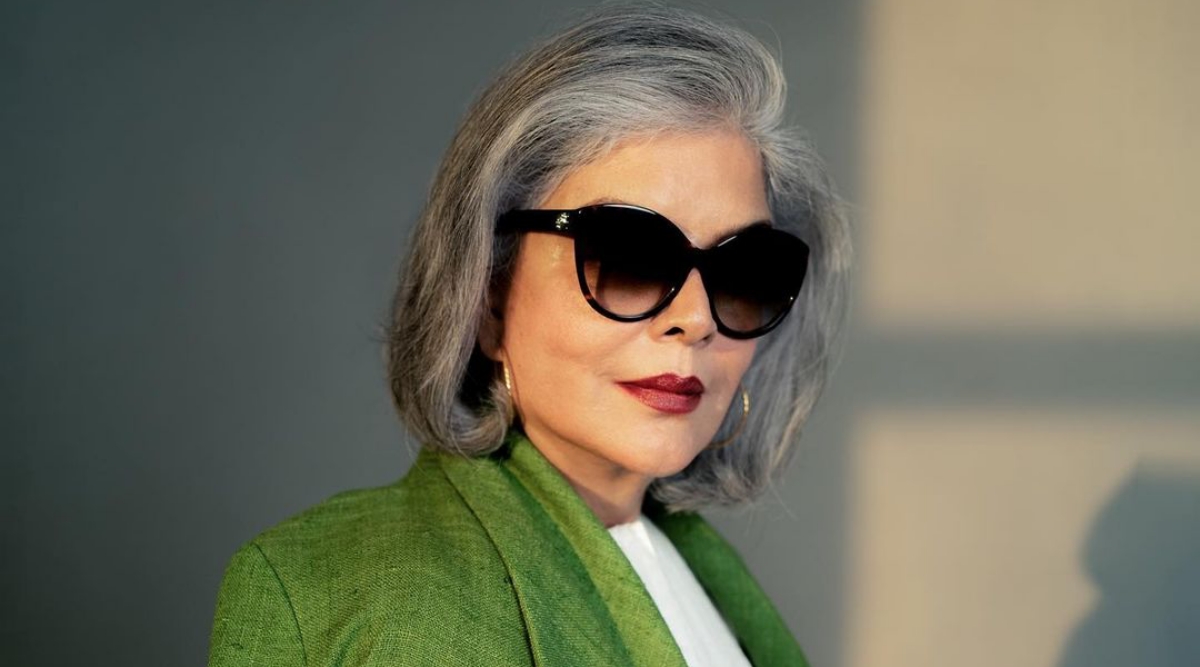In this professional photograph, a distinguished and fashionable mature woman stands confidently against a plain gray backdrop. She is illuminated by a light source that casts a subtle shadow behind her, emphasizing her as the focal point. She sports large, dark black, beetle-sized sunglasses, framing her tan face, which is complemented by carefully applied makeup and striking dark red lipstick. Her hair, a medium-length mix of light and dark gray, is styled in a bob that is brushed back, subtly curled at the ends. She is dressed in a green blazer over a collarless white shirt, with just the shoulders and parts of her arms visible. Elegant gold hoop earrings adorn her ears, enhancing her sophisticated appearance as she gazes thoughtfully out of frame to the right.